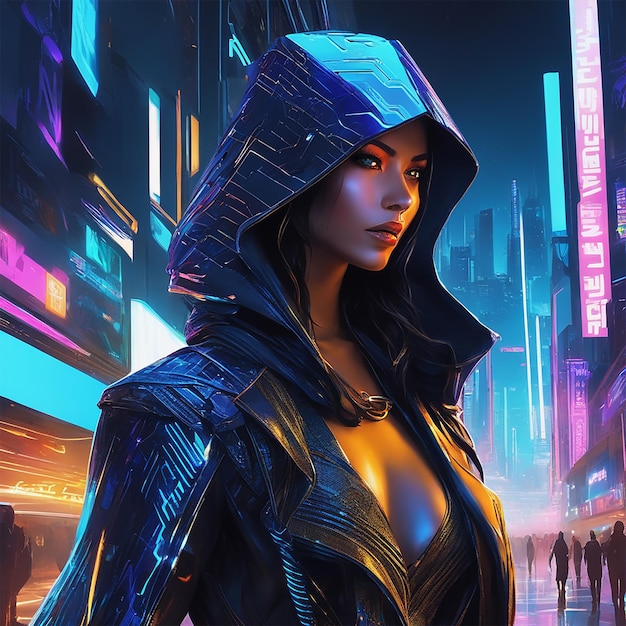The image is a highly detailed digital rendering of a female character, resembling a figure from a video game, set against a vivid cyberpunk cityscape. The woman is depicted from slightly above head level down to below her ribcage. She has striking features with black hair, full lips adorned with red lipstick, and heavy eye makeup. Her gaze is directed downwards to the left, capturing a side profile while allowing both of her eyes to be visible. Her attire is intricate and futuristic: she dons a metallic-looking headpiece with fine lines, dark blue on the sides and light blue on the top, complemented by heavy blue shoulder pads and metallic arm coverings. Her outfit continues with a low-cut, open black suit revealing a necklace around her neck.

Behind her, the city is alive with tall buildings lit by vibrant neon colors characteristic of cyberpunk aesthetics. The background is rich with panels of pink, teal, and light green hues, while sections of fluorescent orange lights cut through a brown area at the lower left. The upper right portion showcases a gradient from light pink to darker pink, adorned with foreign characters in white. Silhouettes of people walk through the city streets in the bottom right corner, adding a sense of scale and life to the scene. The illuminated skyscrapers and neon signs further enhance the city's futuristic ambiance.